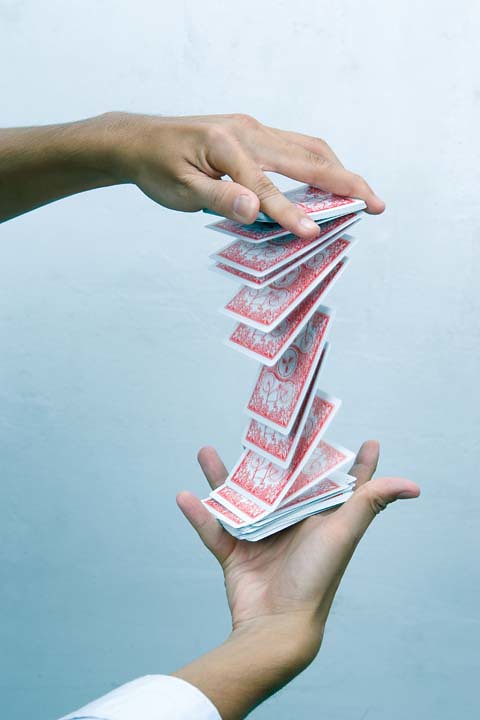In the photograph, a mesmerizing card trick unfolds against a pale blue background. A person's left hand, held high, grips several playing cards that cascade down in a delicate, vertically stretched formation towards their right hand, which is positioned palm-up and ready to receive the falling cards. The image is almost perfectly still, giving the impression that the cards are glued into place, hovering mid-flight. The overall sharpness of the photo lends to the illusion of motion, reminiscent of a flowing waterfall or the elegant pour of wine from a cask. The captivating scene captures both the skill and finesse involved in this intricate display of card handling.